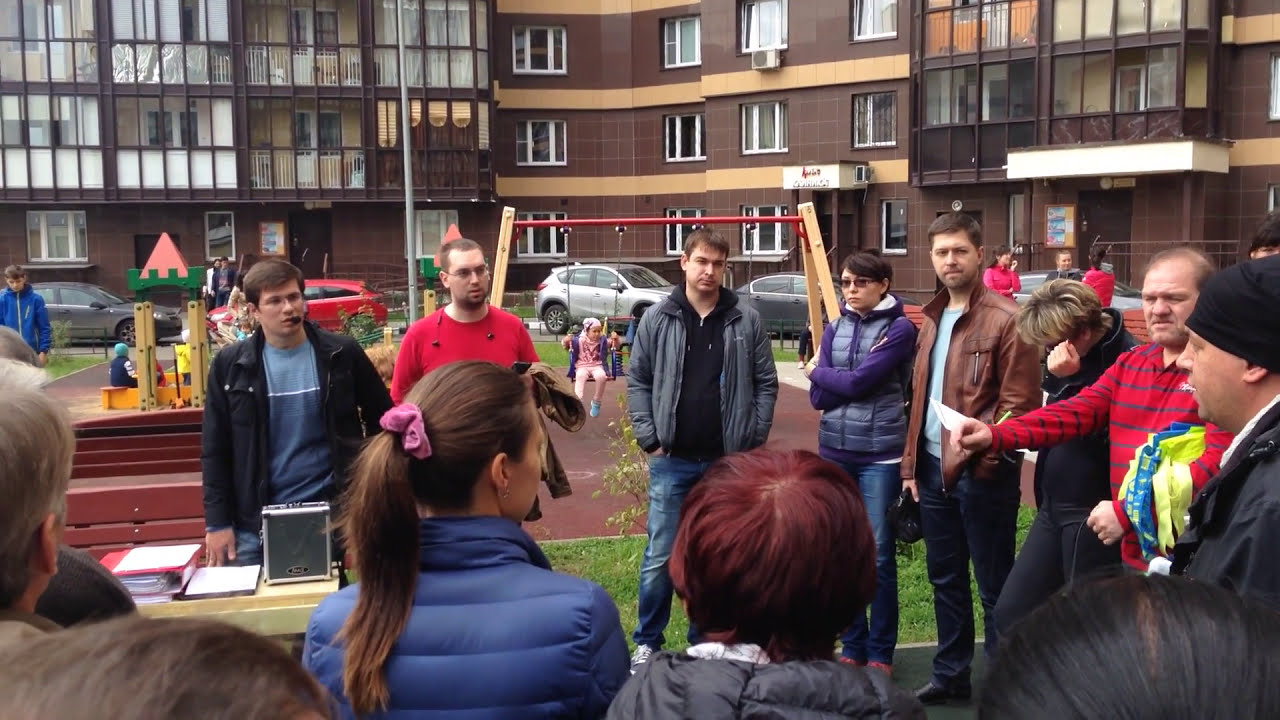In this colorful outdoor scene, a group of 10-15 people is gathered in a circle, seemingly engaged in a discussion. They wear a variety of casual clothing, including jackets, shirts, jeans, and sweatshirts in colors like red, purple, gray, brown, and blue. Visible to the left side of the circle, one person, possibly the leader, stands next to a table with binders and has a small headset microphone. This individual, distinguished with a red shirt with blue stripes and some light green and blue ribbons, gestures with his right hand, possibly emphasizing a point.

Directly behind the group is a vibrant playground, featuring a tan, green, and pink structure. A brown and red swing set with a blue swing adds color, where a girl in a pink shirt is joyfully swinging. Further back, several cars in hues of black, red, and gray are seen moving along a road. The backdrop of the image consists of an apartment complex with brown and tan buildings, accented with white and darker brown trim. The entire scene suggests an organized outdoor meeting or event in a community space.